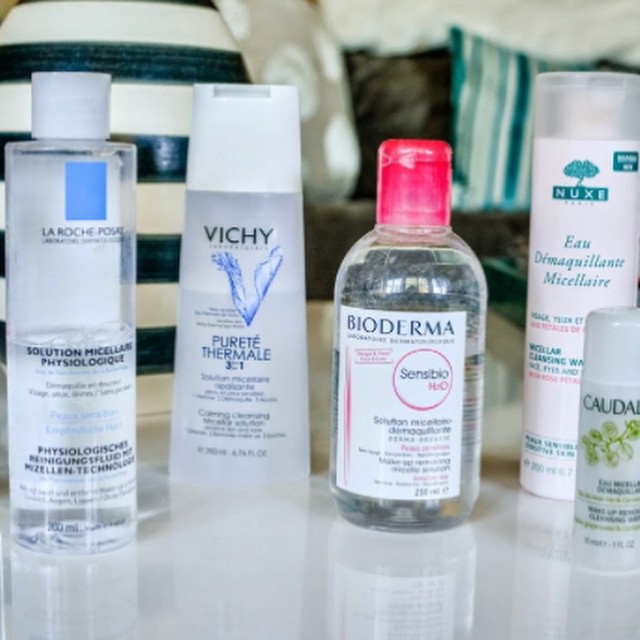The image showcases an arrangement of various toiletry bottles standing on a glossy white counter, their reflections clearly visible on the surface. In the foreground, from left to right, the first bottle is a clear container from La Roche-Posay, identified by its signature blue square logo and labeled "Solution Micellar Physiologiste." The bottle is half-filled with a clear liquid. Next is a three-quarters full clear bottle from Vichy, featuring an image of liquid on the label and marked "Purité Thermal," with the rest of the text too small to discern. Following this is another clear bottle capped in red from Bioderma, bearing a red circle with the words "Sensibio H2O" and more unreadable text. Beside it stands a white bottle from Nuxe, labeled "Eau de Maquillante Micellar." The final bottle, partially cut off from the frame, is white with green leaves and includes the visible letters "C-A-U-D-A," hinting it might be a product from Caudalie.

In the background, a white container adorned with dark green stripes can be seen. Further back, there are blurry pillows, including a black pillow and a green and white striped one. The background also contains dark, indistinct objects that might be furniture, along with another white possibly-furniture element behind the pillows, adding depth and context to the scene.